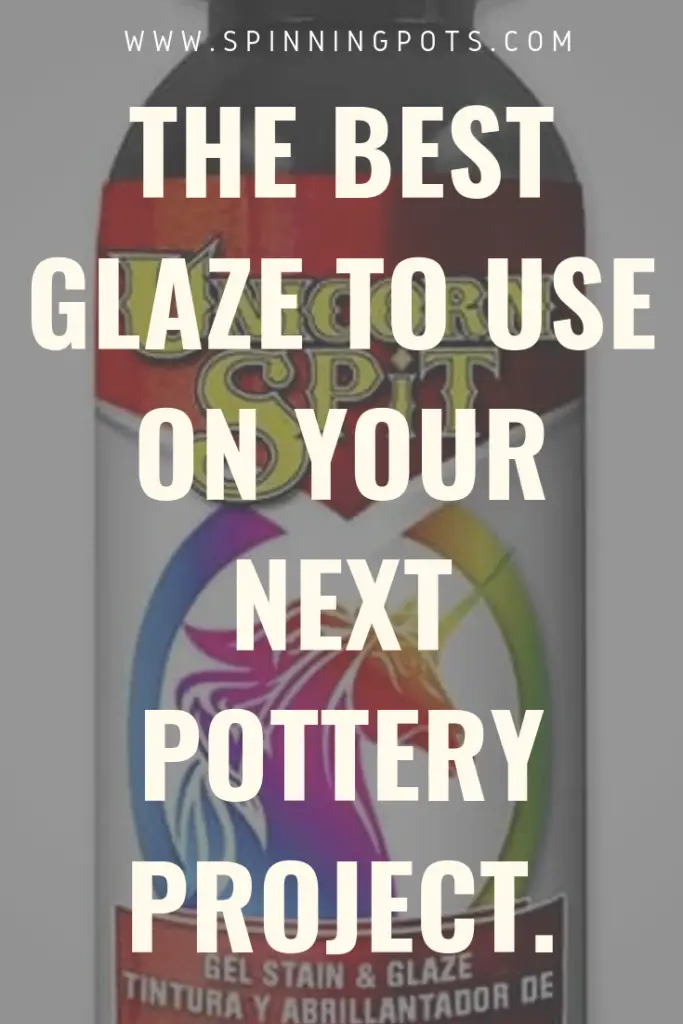At the top of the image, in small white capital letters, is the website www.spinningpots.com. Below it, in large, bold white letters, the text reads: "The Best Glaze to Use On Your Next Pottery Project." This text spans almost the entire height of the image. The background showcases a bottle labeled with "Gel, Stain, and Glazed" in white letters, followed by text in another language, likely Spanish. The bottle features a colorful, tie-dye unicorn design with hues of green, rose, pink, purple, blue, orange, and yellow. The unicorn, facing right, is surrounded by two bowed arches forming almost a circle. Above the unicorn is the product name, partially readable with the second word being "Spit" in yellow letters. The design includes a red rectangular background at the bottom and a smaller red upside-down triangle. The bottle cap is visible at the top, giving the impression that the viewer is closely zoomed in on the product.